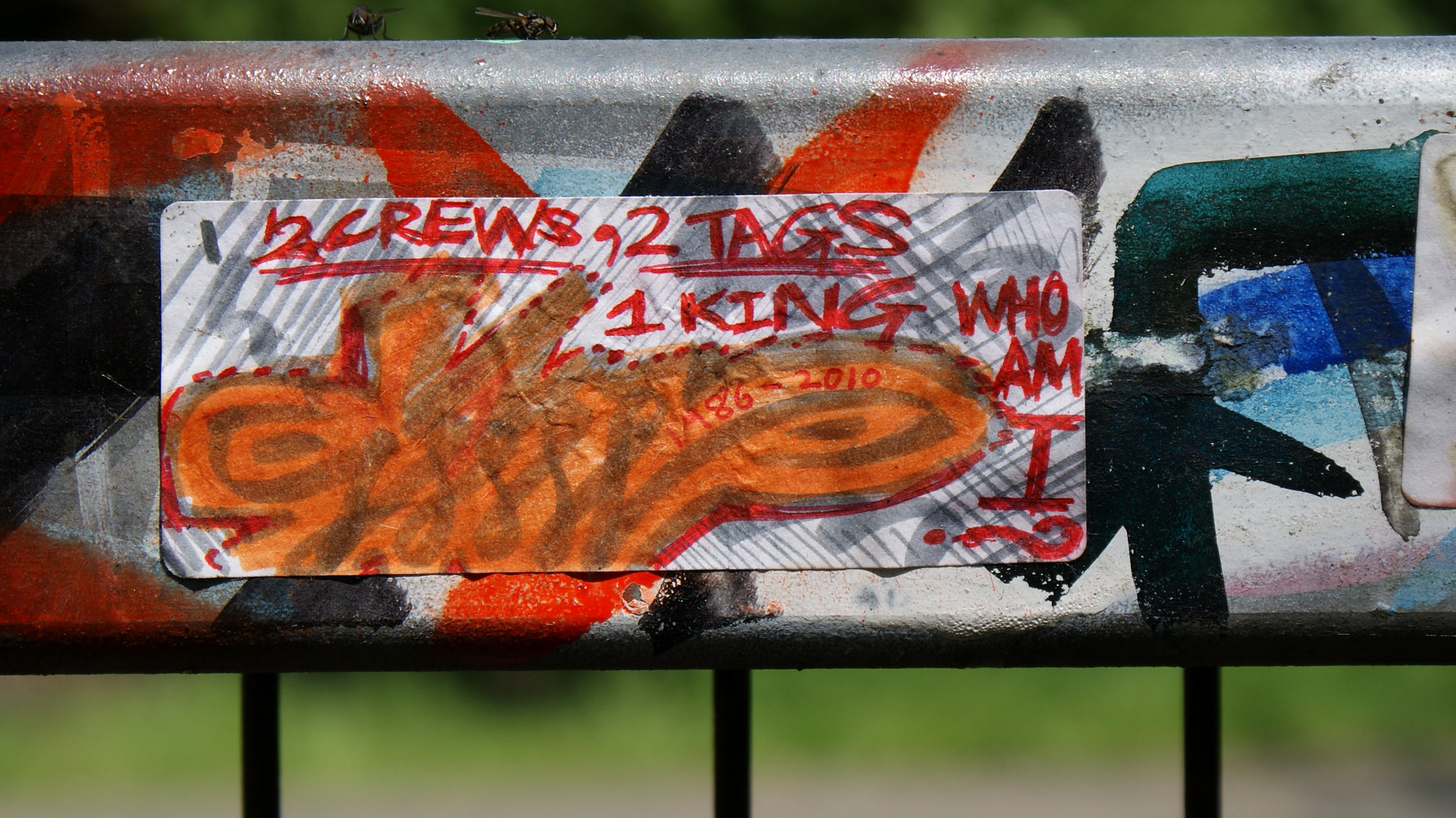This is a high-quality, landscape photograph taken outdoors, depicting a safety rail of a highway covered with layers of overlapping graffiti in various colors including orange, black, blue, dark green, red, and turquoise. The graffiti tags, typical in letter shapes, create a vibrant, chaotic canvas on the metal surface of the railing. Embedded in the graffiti are the numbers "V186-2010". Over the various sprayed tags, there is a large rectangular sticker adorned with additional graffiti. The sticker features text written in red marker, which reads: "2CREWS, 2 TAGS, 1 KING, WHO AM I?" The text is formatted with "2CREWS" and "2 TAGS" underlined, followed by "1 KING, WHO AM I?" stacked line by line, ending with a sideways question mark. Additionally, the sticker also contains an orange tag and grayish-green curved lines surrounded by little red dots, making the entire scene a vivid tapestry of street art. Two small winged bugs rest atop the graffitied metal railing, adding a subtle touch of life to the otherwise static image.